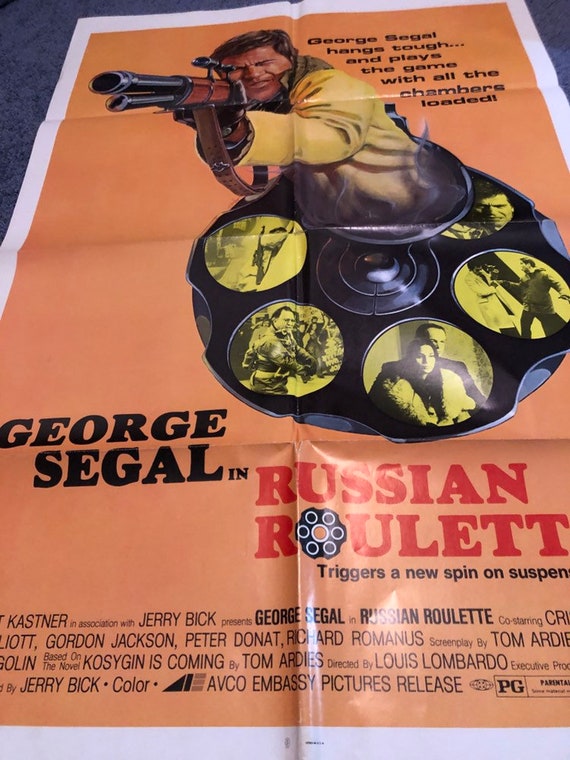This image depicts a detailed but worn poster for the movie "Russian Roulette," which appears to have been folded and smoothed out to the best of someone's ability. The poster features an orange background with black and red text. The title "Russian Roulette" prominently uses a gun chamber illustration for the O, symbolizing the movie’s suspenseful themes. The tagline, "George Segal in Russian Roulette triggers a new spin on suspense," is partially visible, with "suspense" being cut off.

A detailed illustration of the lead actor, George Segal, holding a rifle, dominates the poster. He is depicted emerging from what looks like the chamber of a gun, with different stills from the movie in place of bullets. Another tagline at the top right reads, "George Segal hangs tough and plays the game with all the chambers loaded."

The bottom of the poster lists the movie credits, including the cast—George Segal among them—and mentions that it is based on the novel "Kosygin is Coming." The production and distribution details indicate it’s an Embassy Pictures release, rated PG. The style of the photograph suggests it was taken at an angle, either on the floor or a bed, further emphasizing the poster's worn condition.